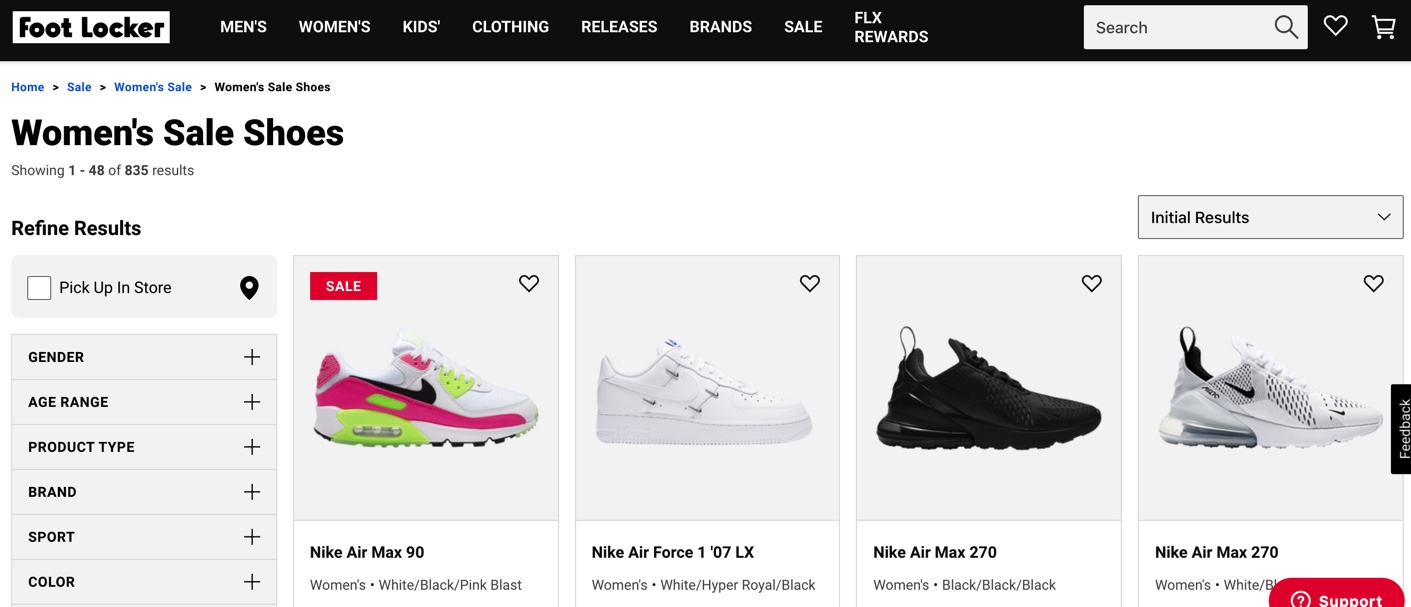The Foot Locker website is prominently displayed, showcasing a well-organized e-commerce layout for an optimal shopping experience. At the top of the page, there are navigational tabs allowing users to explore various categories, including Men’s, Women’s, Kids, Clothing, Releases, and Brands. The site also highlights their “FLX Rewards” program, indicating a loyalty rewards system for frequent shoppers.

On the left side, a refining options panel allows customers to filter results by criteria such as store pickup availability, gender, age, and other specific preferences. To the right, the main display shows initial search results with a drop-down menu for further customization.

Currently featured are four items, all from the Nike Air Force collection, specifically targeting women. Among them, one item stands out as it’s marked on sale: the Nike Air Max 90, showcasing a vivid color combination of pink, lime green, and white, enhanced by a black Nike emblem. The other items include a classic all-white pair, an all-black pair, and a predominantly white pair with subtle black detailing.